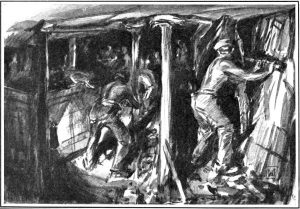This detailed black and white drawing, seemingly a sketch, appears to date back to the early to mid-1900s and depicts a labor-intensive scene, possibly set in a coal mine or similar industrial environment. The medium used is either pencil, black ink, or charcoal, emphasizing the interplay of light and shadow. The setting is enclosed, with a prominent central pillar and several beams extending from the ceiling to the floor, suggesting a confined workspace. 

The image focuses on a group of working men, with their backs towards the viewer. On the left side, there seems to be a drawer or bin, with a couple of men possibly placing something inside. To the right, a partially shirtless man, distinguishable by his cap and glistening skin, appears to be interacting with the wall, either hanging or chipping away at something. Despite its small size and intricate details, the illustration compellingly captures the essence of the labor depicted, leaving much to speculate about their exact activities and the conditions of their work environment.